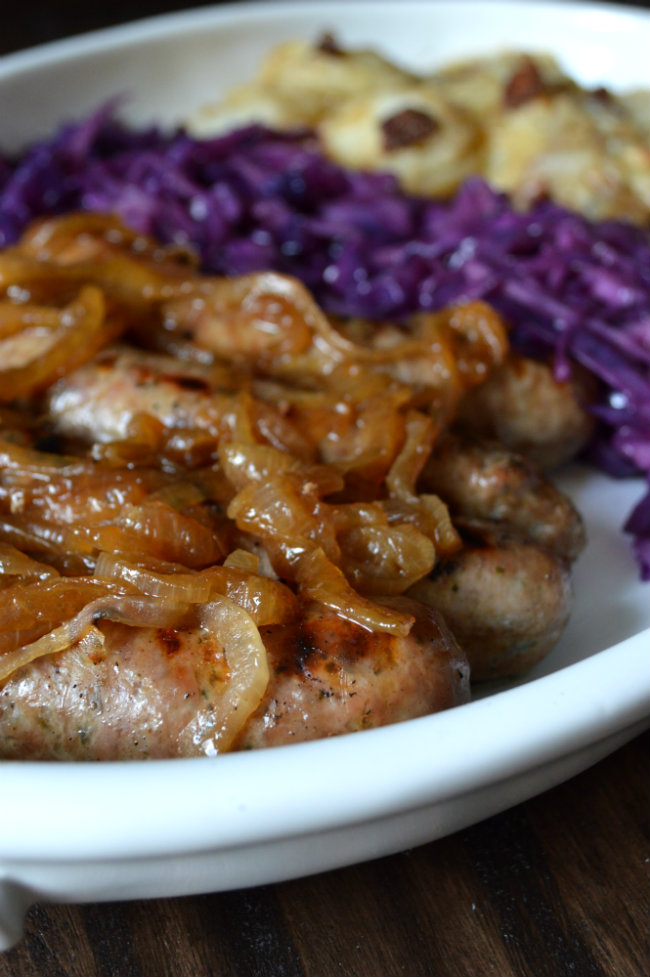This is a close-up photograph of a white porcelain plate sitting on a dark brown wooden table. The plate has a high, smooth edge with a subtle lip, giving it an elegant appearance. The food presentation is divided into three main parts. Closest to the viewer, four brown grilled sausages are neatly arranged with a generous topping of golden sautéed onions, taking up roughly half of the plate. Adjacent to the sausages is a narrow section filled with vibrant, deep purple cabbage, which appears to be boiled and seasoned, its wilted texture suggesting it’s fully cooked. Furthest from the viewer, towards the back of the plate, there is a slightly out-of-focus portion that appears to be mashed potatoes sprinkled with pieces of bacon. This elaborate dish showcases a hearty, well-rounded meal.